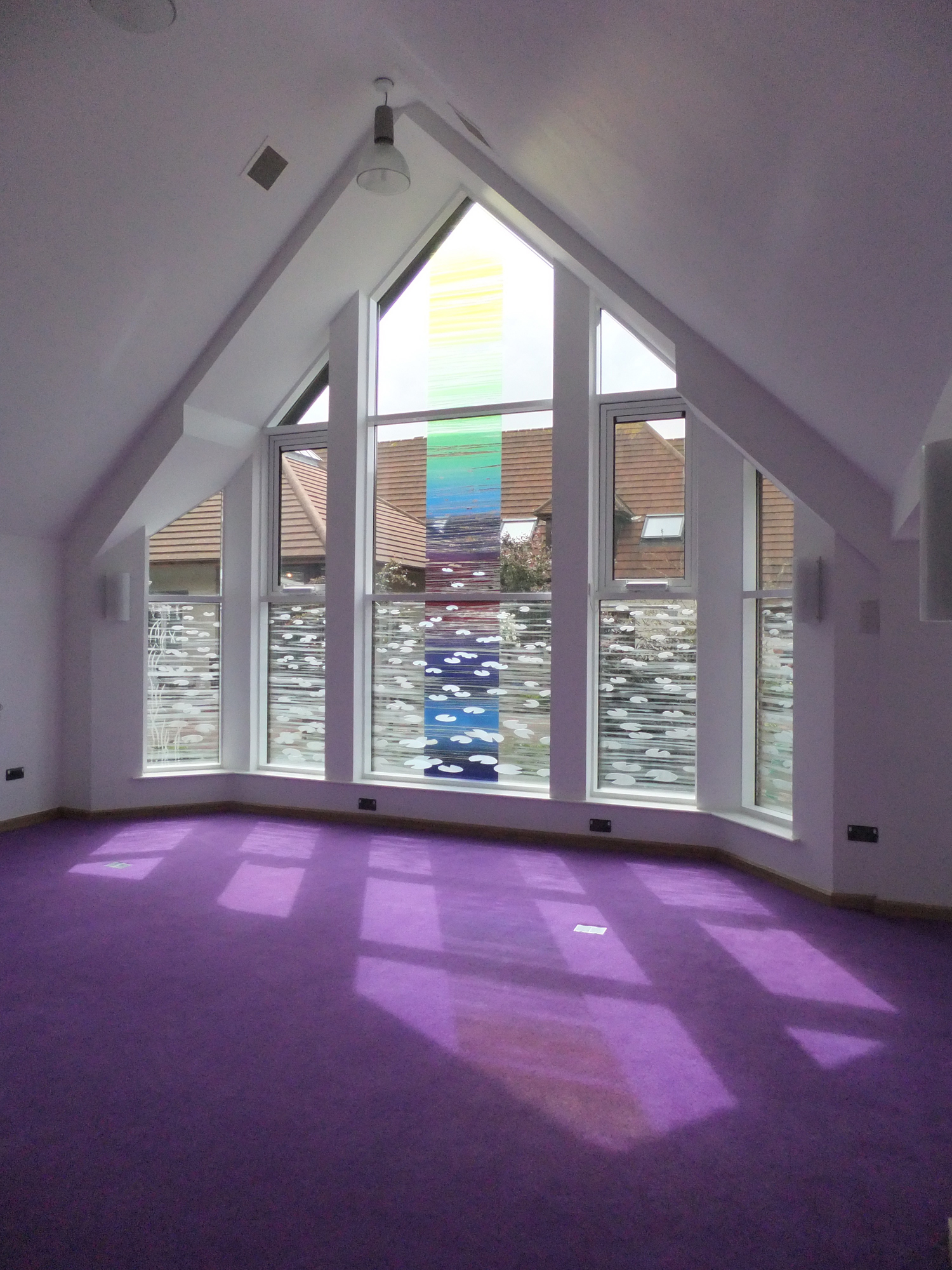The image showcases an interior space that appears to be a room at the top of a building, possibly a church or another type of structure. The room is notable for its distinctive purple floors and white ceilings and walls. Prominently featured is a large, triangular window that allows light to flood the room, casting reflections on the purple surfaces. This window is divided into sections, with the top adorned by a colorful design featuring various hues—yellow, green, blue, purplish red, dark blue, and light blue—while the bottom half has intricate patterns that obscure a clear view of the exterior.

Inside the room, there are two unlit lights hanging from the ceiling. Additionally, a fan is mounted on the top left. On the floor, a piece of paper is visible. Along the top edge of the room, another light fixture is positioned in the left corner. Flanking the window are two lamps, one on each side. Through the window, the roof of an adjacent building with a brown roof and some vegetation is visible, adding to the picturesque view.